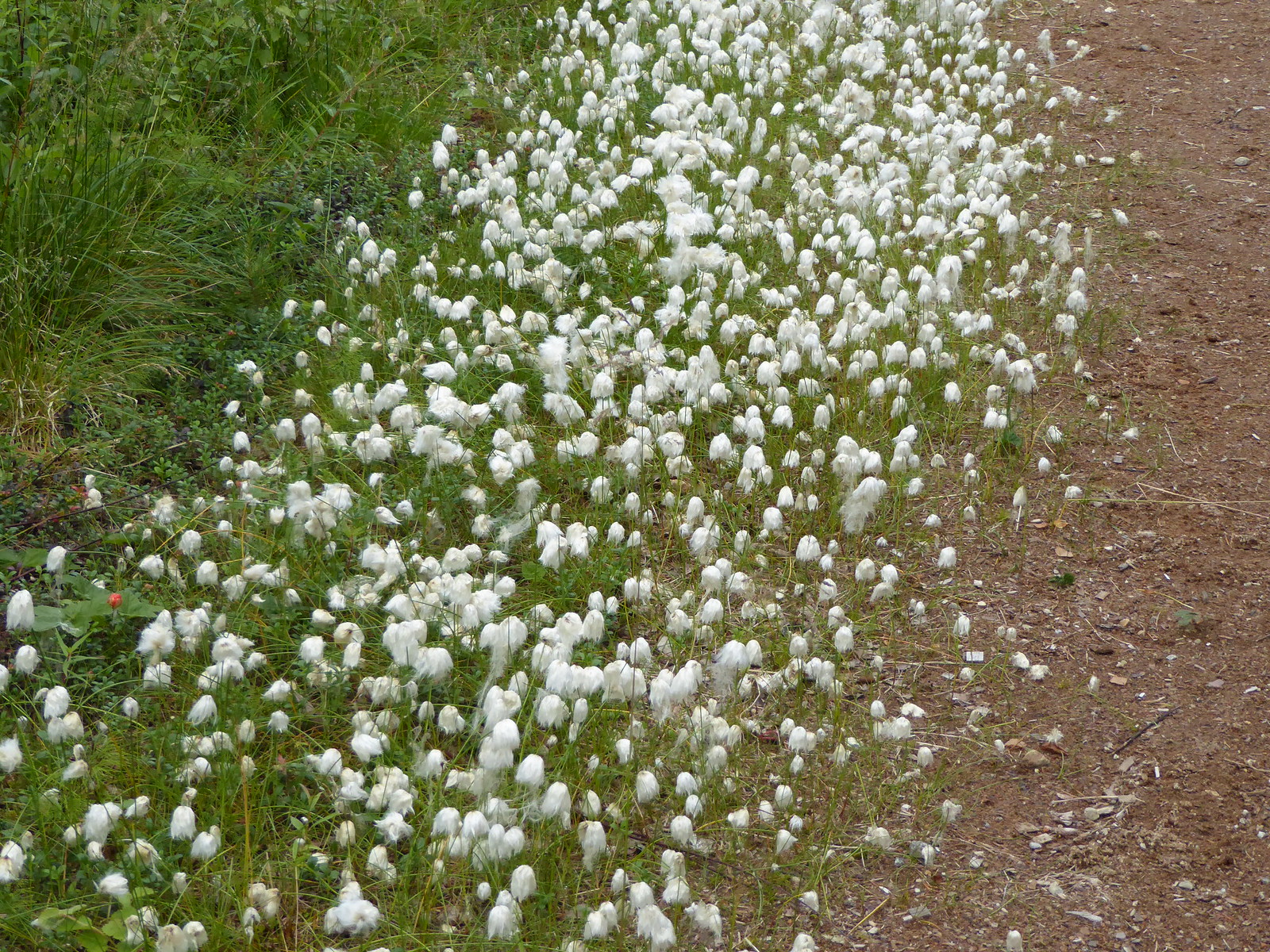This photograph captures a patch of white flowers densely clustered amid a grassy area. The flowers emanate from a lush green patch of stems and grass, creating a striking contrast with their pure white petals. On the left side of the image, taller grasses and weeds tower over the shorter grass that dominates the scene. To the right, a reddish dirt area interspersed with bark chips subtly transitions into the greenery, adding a distinct texture to the landscape. These flowers, resembling a scattering of popcorn, appear in various stages of bloom, with some looking like delicate cotton balls or feathery domes. The scene is further enriched by a red ladybug with black spots perched on a leaf, and a brown butterfly with black wing markings resting on one of the flowers. The photograph lacks other objects or animals, focusing entirely on the natural elements, especially the countless white blooms that resemble a mix of popcorn and hailstones scattered across the green expanse.